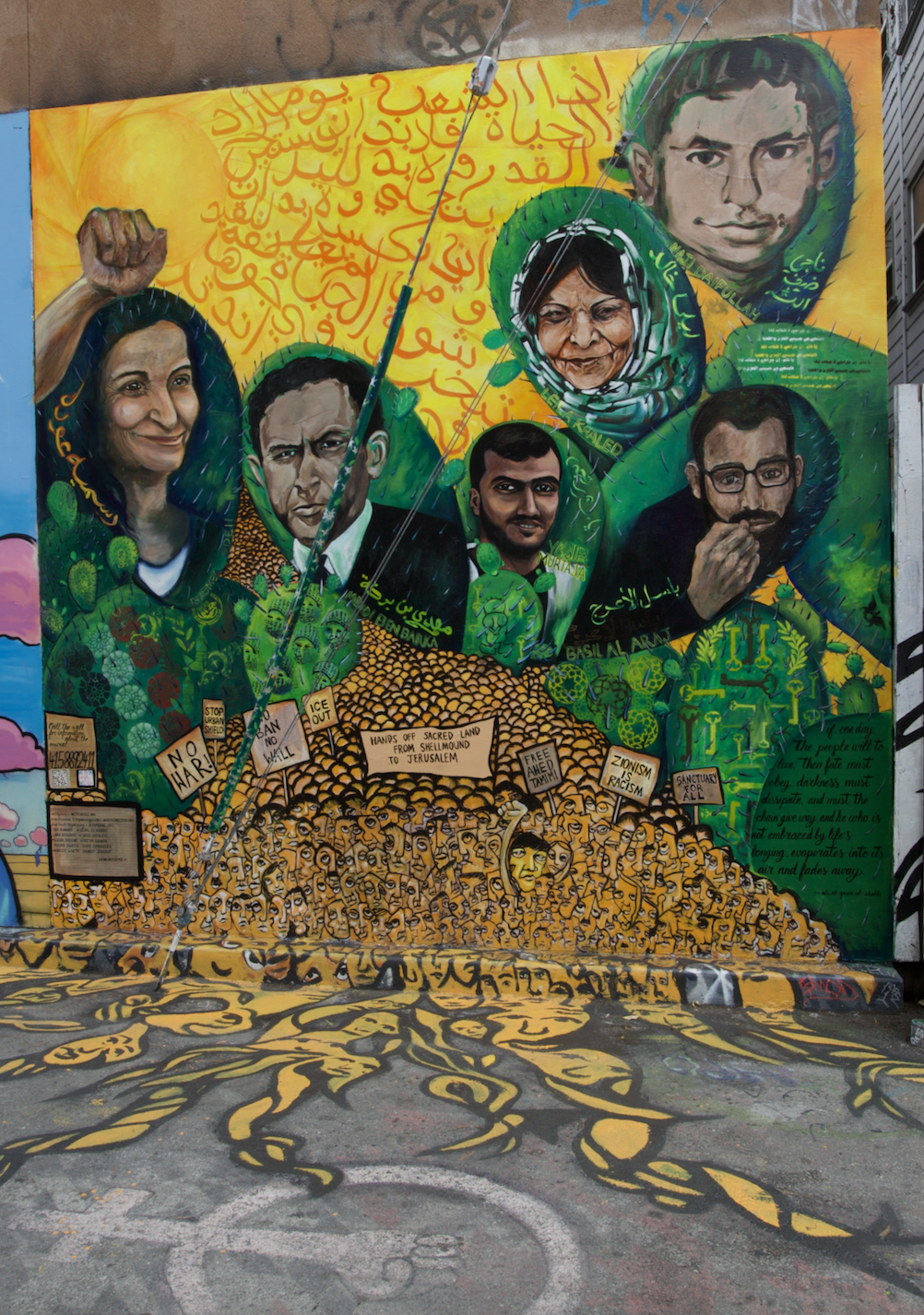The mural, vibrant and politically charged, stretches across a wall and bleeds onto the curb and ground. Dominated by a yellow background with green elements, the mural features six prominent figures suggesting diverse backgrounds, possibly Muslims, given the darker skin tones and the presence of traditional attire like the Palestinian shawl. On the leftmost side, a woman with her fist raised in a triumphant gesture smiles, while next to her stands a man with black hair in a white collar, identified by the name Ben Bajuka. Another man, sporting a dark beard and mustache, appears nearby with the possible name "ORIA" inscribed below him. The mural also includes a bespectacled man with a black beard and mustache, hand raised to his nose, seemingly identified as "BASILALARJ". Above these four figures, two more faces are visible: a woman adorned with a Palestinian shawl and an unreadable name, and a younger boy whose name might end in "PULLAH". The mural’s backdrop is covered with a multitude of smaller faces and proclamations stating, “No war, no ban, no wall, ICE out, hands off sacred land from Shelmon to Jerusalem, free Ahmed Tamimi, Zionism is racism, sanctuary for all.” This scene likely represents a revolutionary gathering or homage to martyrs, conveying resounding anti-war, anti-racism, and pro-human rights messages.